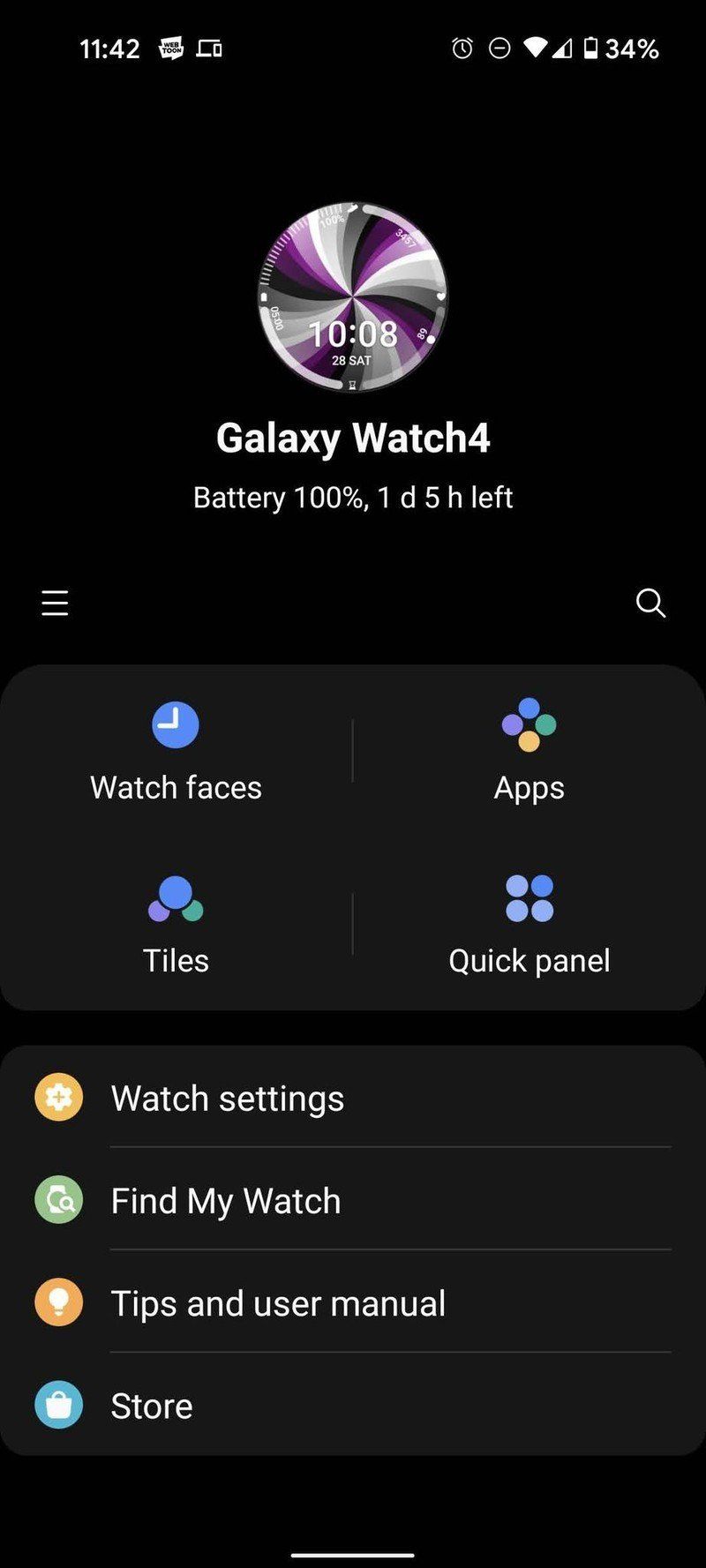This image depicts a smartphone screen displaying a user interface with detailed information and options for a connected Galaxy Watch 4. The phone shows the current time as 11:42, with a battery level of 34%, and a decent signal strength. The screen is set against a black background, creating a stark contrast that highlights the vibrant elements on the display.

Prominently featured is an icon representing a CD with mesmerizing swirls of purple, silver, and white, adding a touch of elegance. The Galaxy Watch 4 information is clearly presented, showing a full 100% battery with an estimated life of one day and five hours remaining.

Additionally, the interface allows users to alter watch faces. This functionality is symbolized by a circle displaying a clock icon. Various other options are lined up neatly in the display: 

- Watch settings, indicated by a yellow circle containing a settings icon.
- "Find My Watch" feature, symbolized by a green circle with a magnifying glass and watch face.
- Tips and user manual, represented by a light bulb in an orange circle.
- The store, marked by a blue circle with a purse icon.

Each icon is distinct and color-coded, making navigation intuitive and user-friendly. The overall presentation is clean and visually organized, emphasizing the seamless integration of the Galaxy Watch 4 with the smartphone.